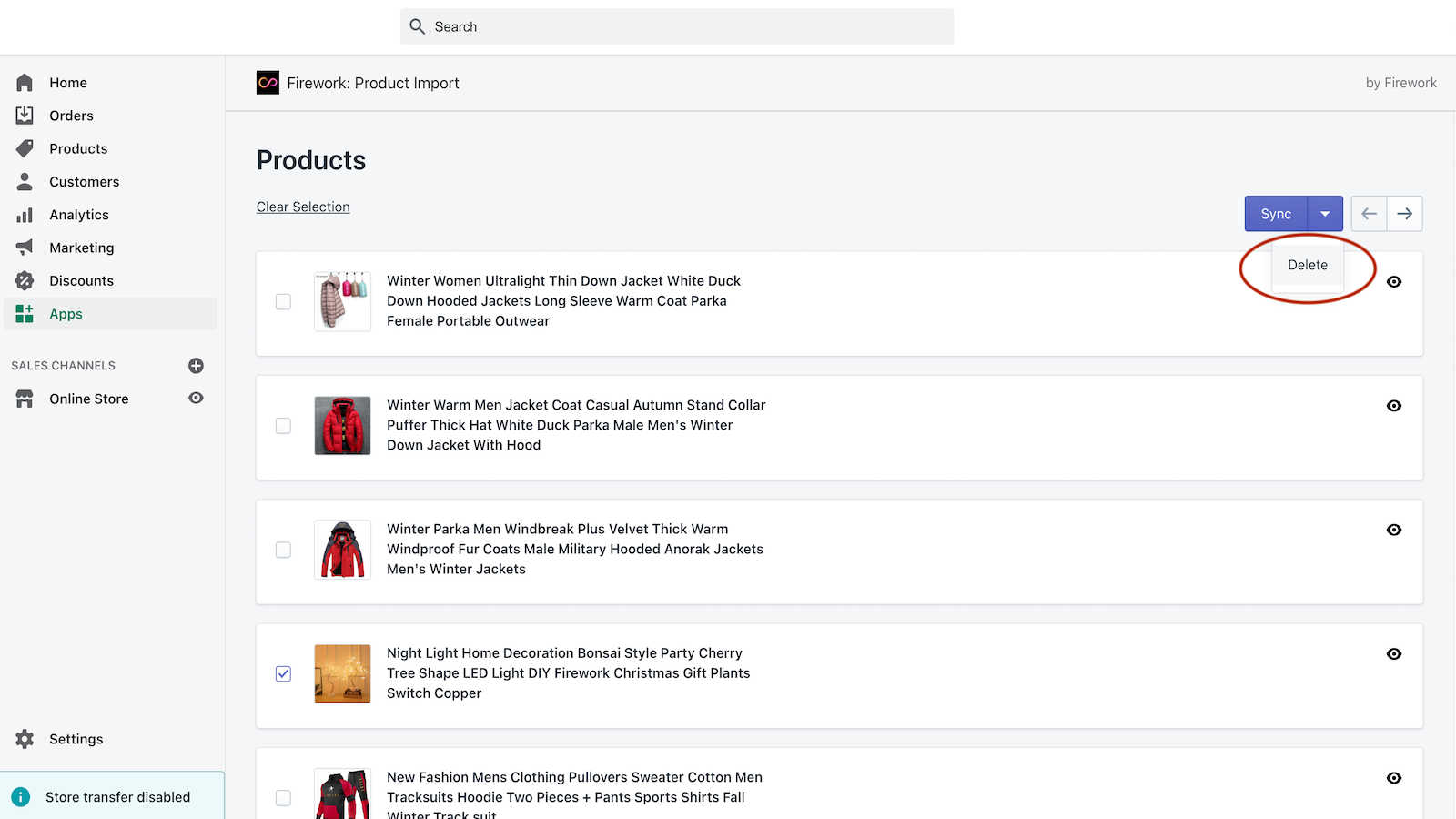This image appears to be a detailed screenshot of a product-based e-commerce website interface. 

At the top right corner, the text "Buy Firework" is displayed in light grey. Centrally positioned at the top is a search bar, prefixed with the word "Search" and a magnifying glass icon to the left. To the left of the search bar, there is a navigation menu starting with the word "Home" accompanied by a home icon.

The left sidebar menu lists various options in a vertical arrangement starting with "Orders" followed by "Products," "Customers," "Analytics," "Marketing," "Discounts," and "Apps." Further down, there is a section labeled "Sales Channels," under which is the "Online Store" option. At the bottom left of the sidebar, there are "Settings" and "Store Transfer Disabled," with a gear icon adjacent to "Settings."

At the top middle section of the interface, the title "Firework Product Import" is displayed, accompanied by a small black square indicating an active status (possibly titled "side 8"). Underneath this title, the label "Products" is prominent, followed by a list of five products. These products are:

1. Winter Women Ultralight Thin Down Jacket White Duck
2. Winter Warm Men Jacket
3. Winter Parka Men Windbreak
4. Night Light Home
5. Pullover Sweater